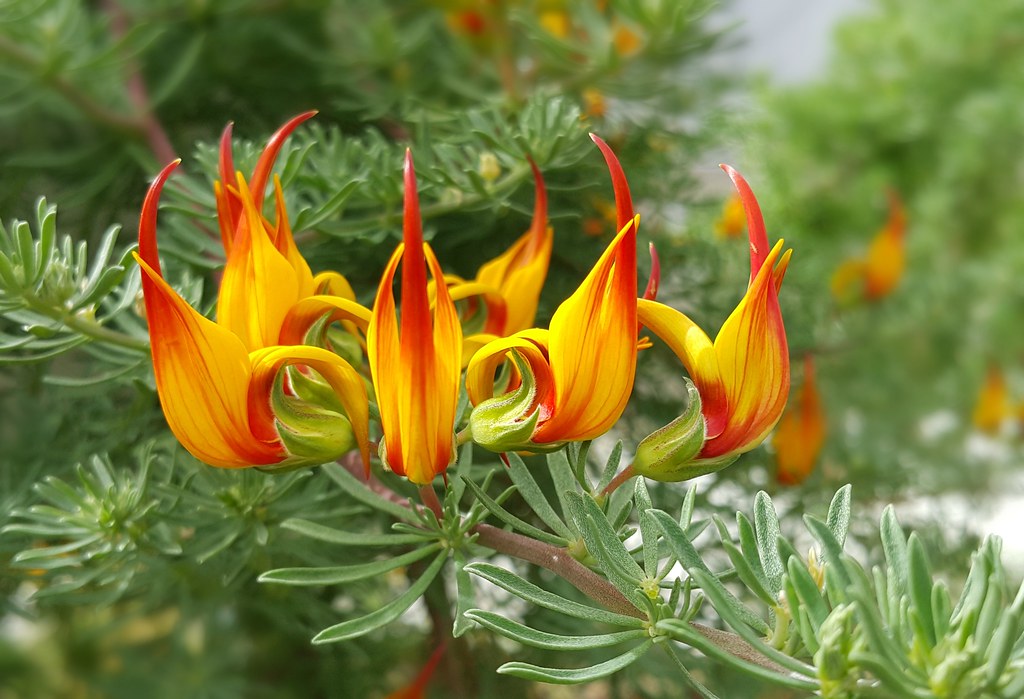This detailed close-up photo features a striking floral arrangement with vibrant yellow flowers accented by red and orange tips. The flowers, which resemble bulbs that have just popped, are partially or not fully bloomed, revealing their colorful inner petals despite their unopened centers. Multiple flowers cluster together on the plant's thick stem, surrounded by an abundance of long, skinny, green leaves that radiate in every direction, reminiscent of star shapes. The background is filled with additional indistinct clusters of similarly colored, unbloomed flowers and numerous green pine branches. As the image extends further back, the focus softens, revealing a blurred scene of more green foliage and pine trees. The overall impression is of a lush, blooming grove, capturing the vibrant and rich detail of the near flowers in striking contrast with the softer, verdant surroundings.